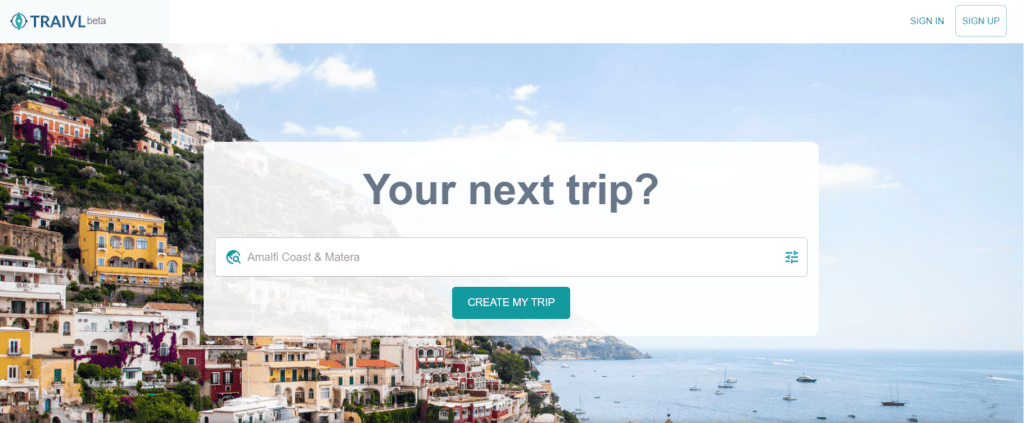This image features a website banner with multiple sections and a scenic outdoor background. Across the top part of the banner, there is a small pale blue box containing the word "TRAIVL" in uppercase dark blue letters, followed by the term "beta" in smaller lowercase letters. To the right side of the top section, there are links for "sign in" and "sign up" in blue print, with "sign up" enclosed within a square outline.

The main portion of the banner showcases a picturesque outdoor scene. On the right side, a tranquil body of water reflects the blue sky, which is adorned with fluffy white clouds. Several boats can be seen floating on the water. On the left side of the water is a rocky mountain or hilly area dotted with houses in various colors, including orange, yellow, red, white, and tan. This hillside is interspersed with lush green trees and foliage.

Centrally located within the banner is a horizontal band resembling a search engine bar with the text "Your next trip?" followed by the names "Amalfi Coast" and "Matera." Beneath these names, the phrase "Create my trip" invites users to plan their journey.